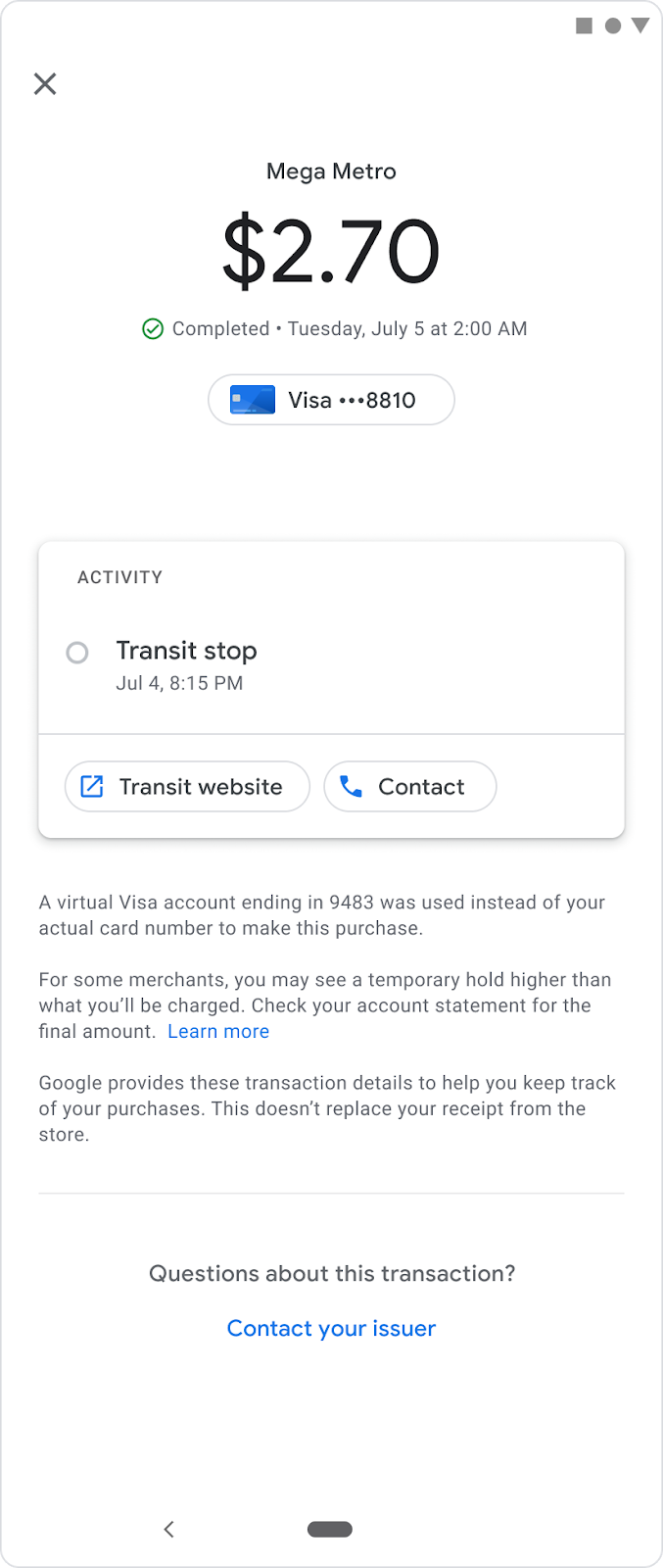**Caption:**

This screenshot, taken from a mobile payment app, showcases a completed transaction with the transit service provider Mega Metro. The image, displayed in a vertical aspect ratio appropriate for mobile devices, details a transaction of $2.70 made using a Visa card ending in 8810. The payment was processed on Tuesday, July 5th at 2:00 AM for a transit activity that took place on July 4th at 8:15 PM.

Key features of the screenshot include options to visit the transit service's website or contact them via phone. At the bottom, a disclaimer notes that a virtual Visa account ending in 9483 was used instead of the actual card number for added security. It also mentions the possibility of seeing a temporary hold that may differ from the final charged amount, advising users to check their account statements for the final transaction details. Google provides these action details for better purchase tracking but emphasizes that this information does not replace the receipt from the store. Additionally, there is a contact section at the bottom for users to reach out to the issuer with any questions regarding the transaction.